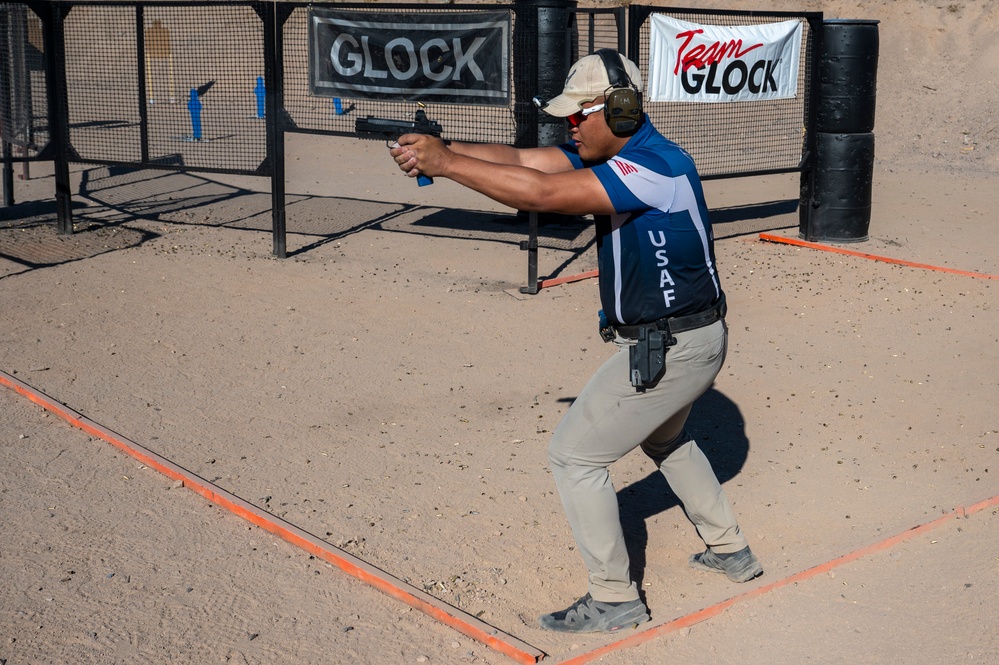In this image, a man is engaged in target shooting at a gun range, standing poised on a white sandy surface enclosed by an orange square perimeter. He is holding a black handgun, with his arms fully extended in front of him, ready to fire. Dressed for competition, he wears a blue short-sleeved shirt emblazoned with "USAF" in vertical letters on the side, featuring white stripes down the front and back. His outfit is completed by khaki pants and black tennis shoes. For ear protection, he sports large earmuffs and a white baseball cap, along with red sunglasses. Attached to a belt around his waist is a gun holster. Surrounding the area behind him, mesh netting forms a fence decorated with signs reading "Glock" and "Team Glock." Additional obstacles and blue human-shaped targets can be seen faintly in the background. The man is caught in action as a bullet casing ejects from his gun, highlighting the intensity of the moment.